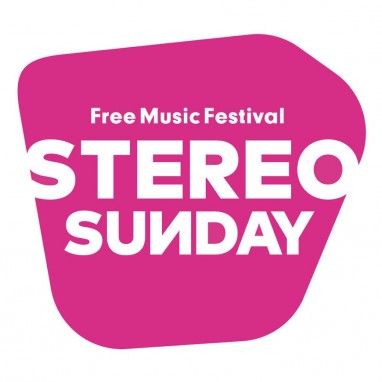The image depicts a vibrant logo set against an all-white background. Dominating the center of the image, the logo is an irregular pentagon shape with five curved corners, broader at the top than the bottom, and colored in a striking hot pink. Within this shape, there are three lines of text, all written in bold white letters. The first line reads "Three Music Festival," with only the initial 'T' capitalized. The second line, "STEREO," and the third line, "SUNDAY," are fully capitalized, with the last letter of "SUNDAY" intriguingly flipped horizontally. The eye-catching design and contrasting colors suggest this logo is likely used to advertise a music festival, perfect for inclusion on business cards, posters, or websites. Both the logo and its text are centrally positioned, occupying a significant portion of the image space.